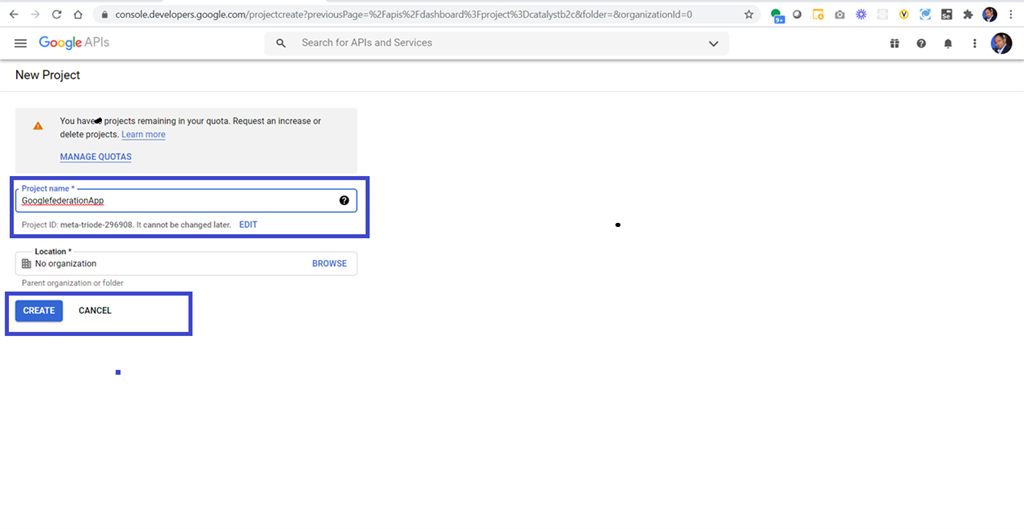The image features a clean, white background with a Google API interface prominently displayed. At the top, there is a functional search bar along with a profile picture icon. Below this, a new project setup section is highlighted. 

A gray rectangle contains various pieces of information, including a yellow notification box with a white exclamation mark, drawing attention to specific details. Adjacent to this are blue links labeled "Learn More" and "Manage Quotas." 

Further down, the image shows a field titled "Project Name" where the project input is displayed. Alongside it is a small black circle with a white question mark inside, offering additional information. 

There is also an "Edit" option in blue, followed by location details and an "Organization" field, which reads "No Organization." A blue "Browse" button and a "Create" button with white text round out the interface options visible in the image.